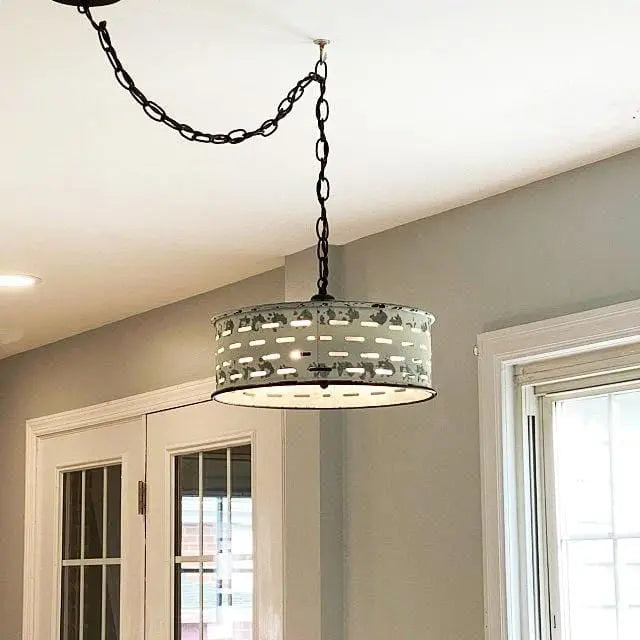This color photograph captures the inside of a house, focusing on an elegant light fixture hanging from the ceiling. The light fixture, reminiscent of a short cylinder or hockey puck in shape, is suspended from a dark gray chain that starts in the top left corner, wraps around a hook to the right, and then descends. The fixture itself has small slits around its edges but primarily emits light from the bottom. Below, on the left, are French doors leading to another room, while on the right, a window with a white frame allows bright sunlight to stream in, illuminating the gray painted walls. Additional ambient light is provided by another ceiling light visible above one of the doors, adding to the overall ambiance of the room.